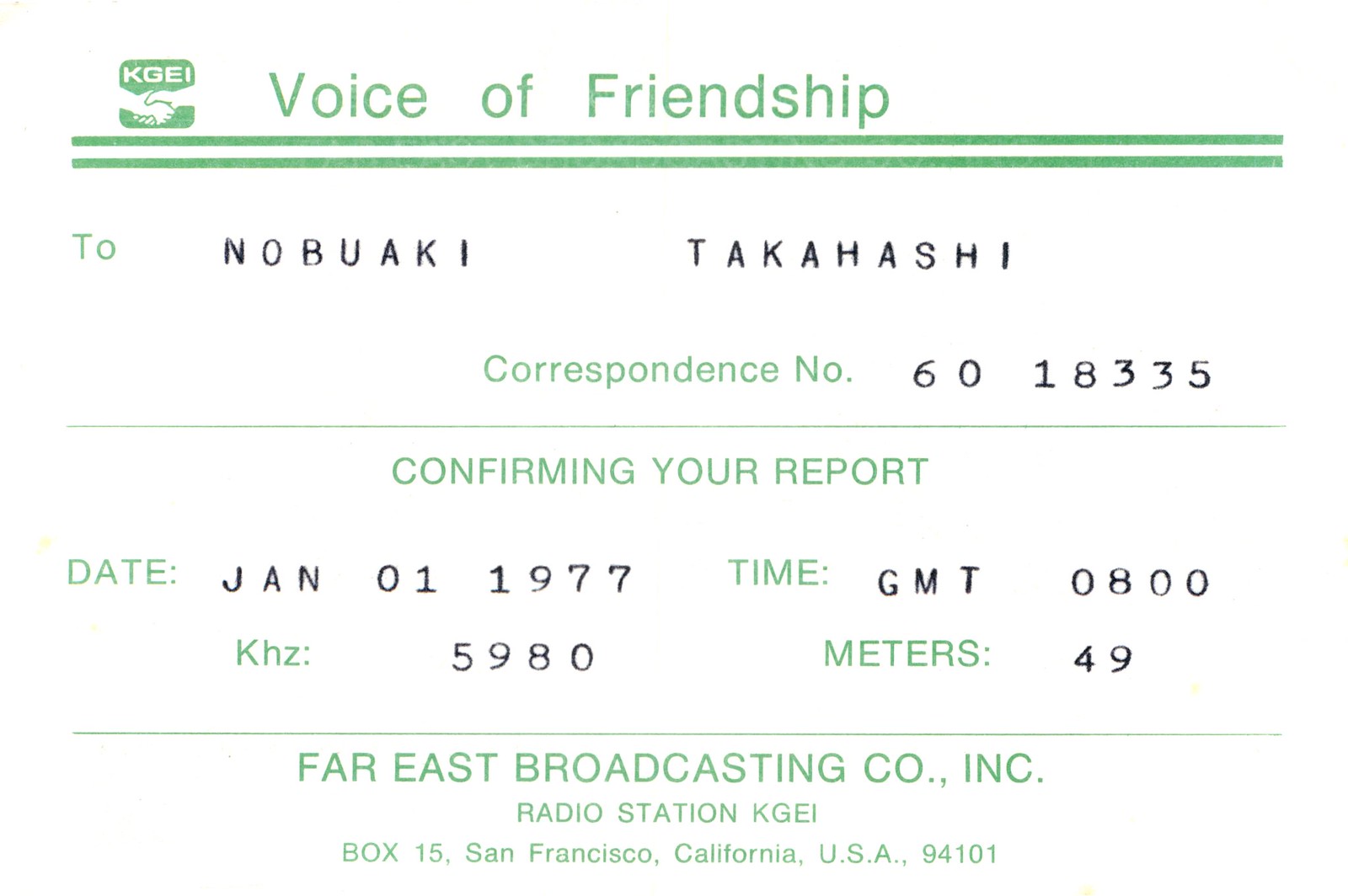The image shows a receipt on a white background with green and black text. At the top, in green text, is "KGEI, Voice of Friendship," accompanied by an icon of two hands shaking. Beneath this, two horizontal green lines separate sections of the receipt. The next section is addressed to Nabuake Takahashi, with a Correspondence Number of 6018335. Further down, the document confirms a report with details: Date - January 1st, 1977, Time - GMT 0800, KHz - 5980, and Meters - 49. At the bottom, it lists "Far East Broadcasting Co. Inc., Radio Station KGEI, Box 15, San Francisco, California, USA, 94101."